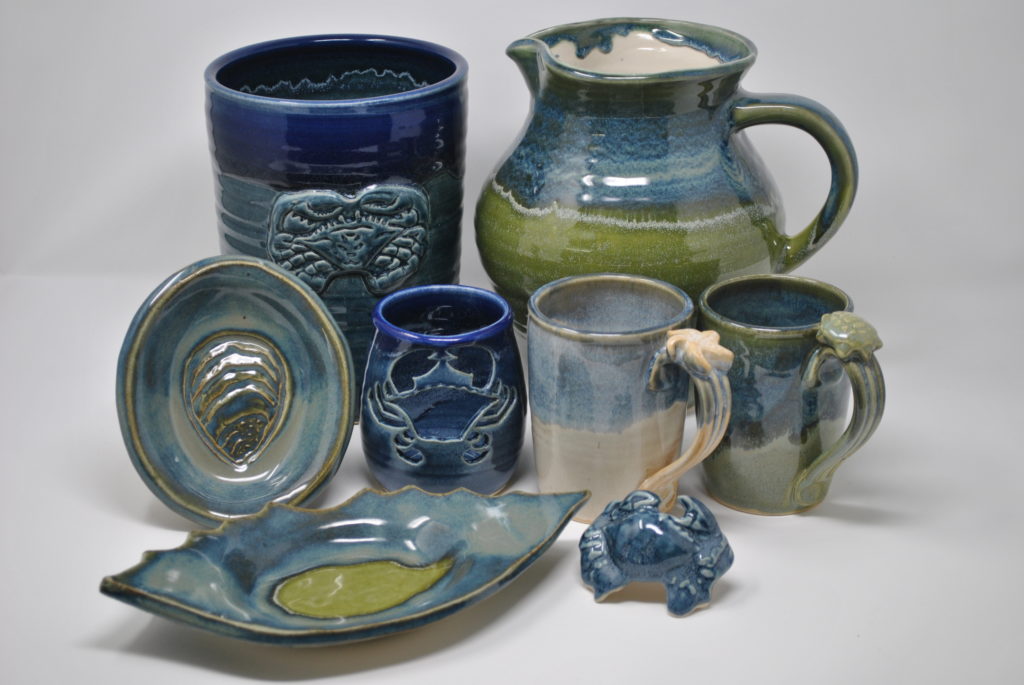This photograph captures an intricately arranged collection of ceramic items with an underlying sea theme. The foreground features an elliptical-shaped serving dish with irregular edges, reminiscent of an oyster shell. Adjacent to it, a small ceramic trinket shaped like a blue crab nestles comfortably. A row comprising a single plate and three cups, all beautifully glazed in varying shades of blue and green, sits beside these items. Each cup is adorned with embossed sea-themed designs, showcasing a turtle, a seashell, and a crab, while the plate features an oyster embossing. In the background, a large blue striped urn stands tall next to a green pitcher, anchoring the collection with their larger presence. The overall arrangement might suggest an old tea set, with its mix of differently sized pieces and maritime motifs, blending functionality with decorative artistry.